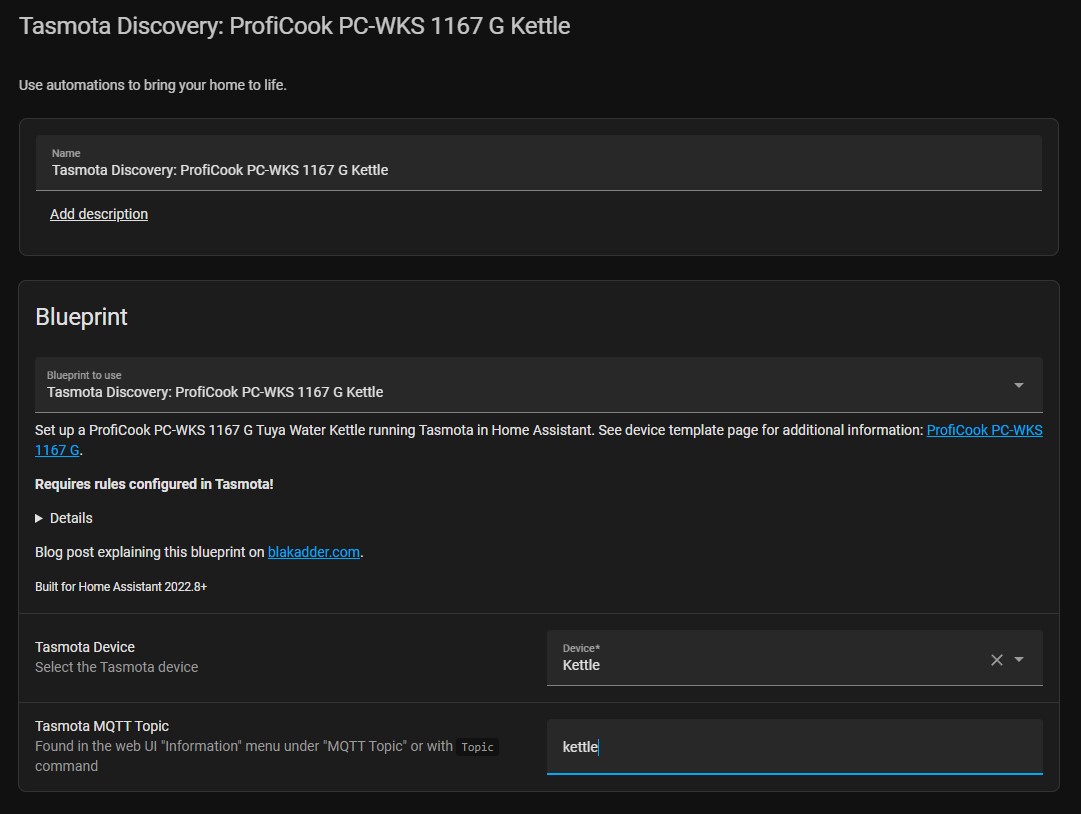Here is a cleaned-up and detailed caption for the described image:

---

The image features a sleek, black and gray background, reminiscent of a dark mode theme. The white text in the upper left corner reads "Tasmota Discovery PROFICOOK PC-WKS1167G Kettle." It encourages users to leverage automations to enhance their smart home experience by introducing the Tasmota Discovery PROFICOOK PC-WKS1167G Kettle. Below this, there is a gray box labeled "Blueprint," which includes a drop-down menu also labeled "Tasmota Discovery PROFICOOK PC-WKS1167G Kettle."

The image guides users on setting up the PROFICOOK PC-WKS1167G TUYA water kettle running Tasmota within Home Assistant. A clickable blue link is provided for the device template page, offering additional information. It emphasizes that rules must be configured in Tasmota. For further details, users are directed to a blog post on blockedter.com. This setup is tailored for Home Assistant version 2022.8 and above, with the specified device identified as a "kettle."

Finally, information about the Tasmota MQTT topic is provided, indicating that it can be found in the web UI under the information menu or obtained using the "topic" command, displaying the topic as "kettle."

---

This caption maintains the original information while presenting it in a clear, structured manner.